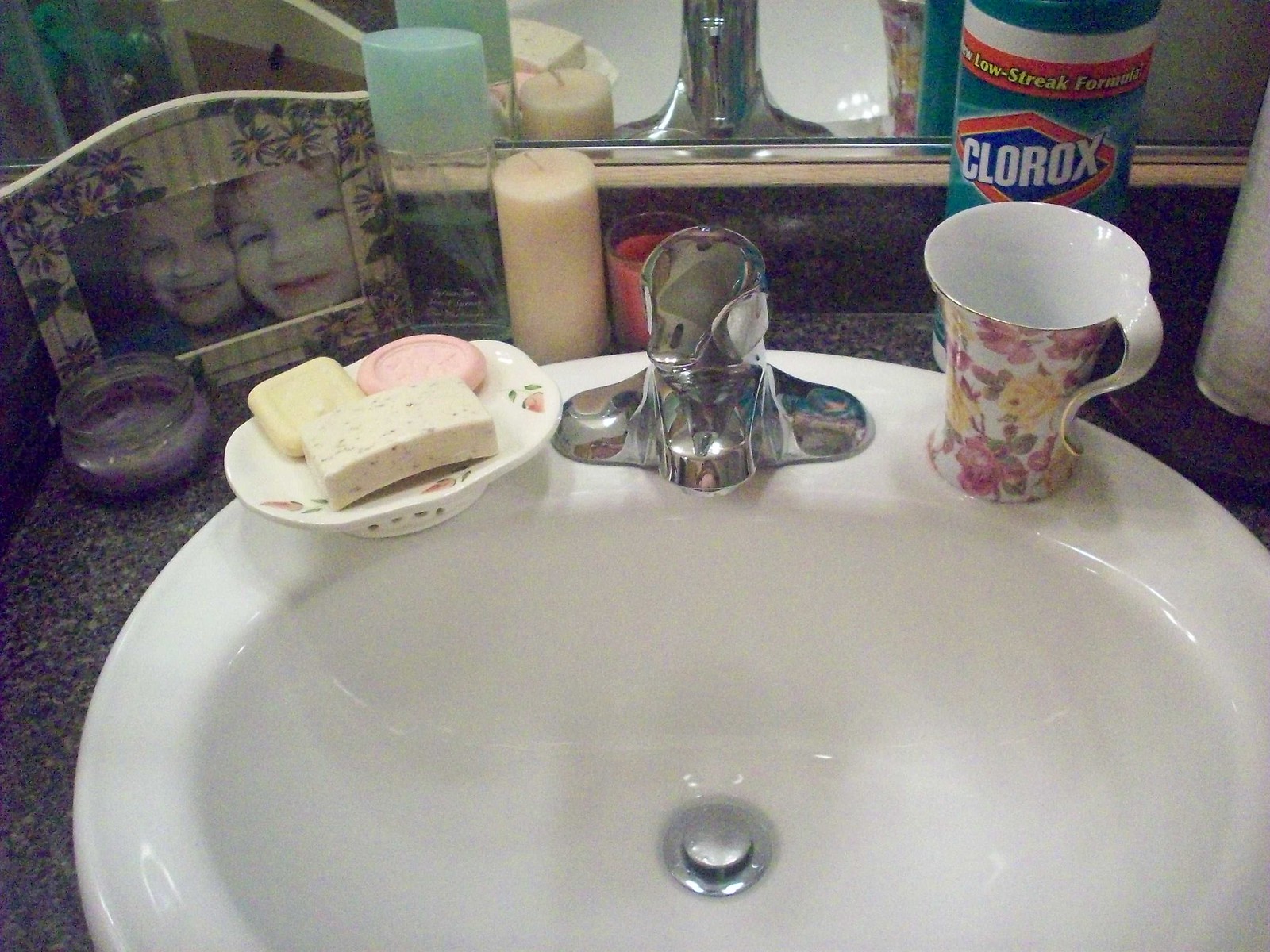The image depicts an old, white bathroom sink, seemingly captured with a low-resolution, pixelated camera. The sink's faucet is centrally positioned, and to its left sits a soap dish holding three differently colored soaps—white, yellow, and pink. To the right of the faucet, there's a glass mug decorated with floral prints. 

Above the sink, a bit of the mirror is visible, reflecting some background items. Positioned at the back of the sink and in front of the mirror is a framed picture of two children, encased in a frame adorned with floral prints. In front of this frame, there's a small purple candle housed in a round jar-like container.

Adjacent to the framed picture on the right is a tube or bottle of perfume, followed by a white candle. Further to the right, there is another candle, this time red. Completing the array, there is a box of Clorox wipes next to what appears to be a roll of paper towels.